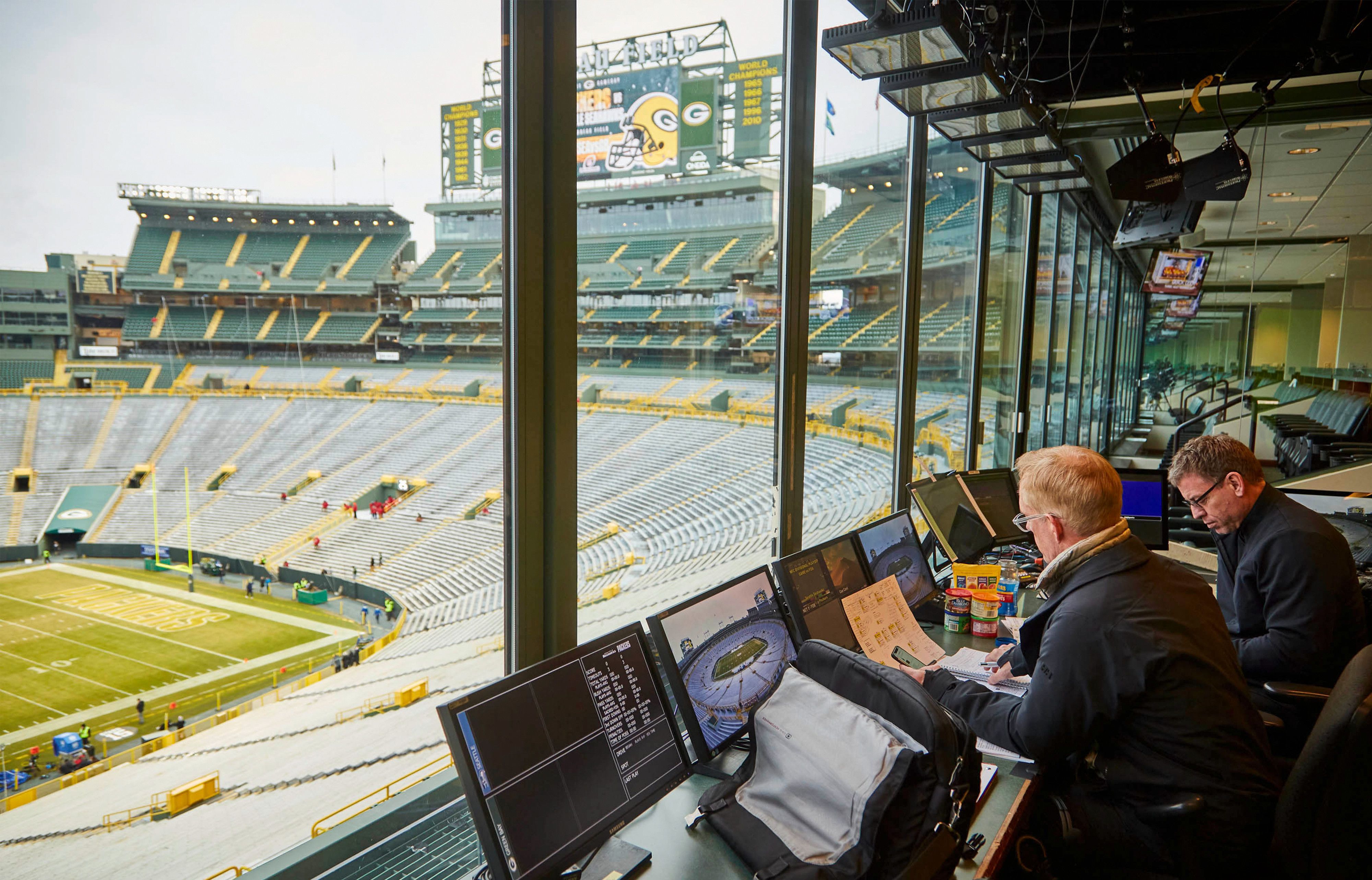In this photograph, we see a detailed view from inside the announcers' booth at Lambeau Field, home of the Green Bay Packers. Through the large glass windows, the iconic green and yellow stands of the stadium are visible, nearly empty as it must be right before the game. The empty bleachers, colored white at the bottom and green higher up, surround the expansive football field where a few indistinguishable individuals are walking. The end zone and a yellow field goal post are clearly visible. Above the stands is a large scoreboard adorned with the Green Bay Packers logo and helmet, signaling the forthcoming game. 

Inside the booth, two announcers, both middle-aged men in dark blue jackets and glasses, are preparing for the game. They are seated side by side, engrossed in their notes and statistics displayed on several computer monitors. The photo captures them from a side profile, emphasizing their focused expressions and the high-tech equipment they use to deliver the game commentary.